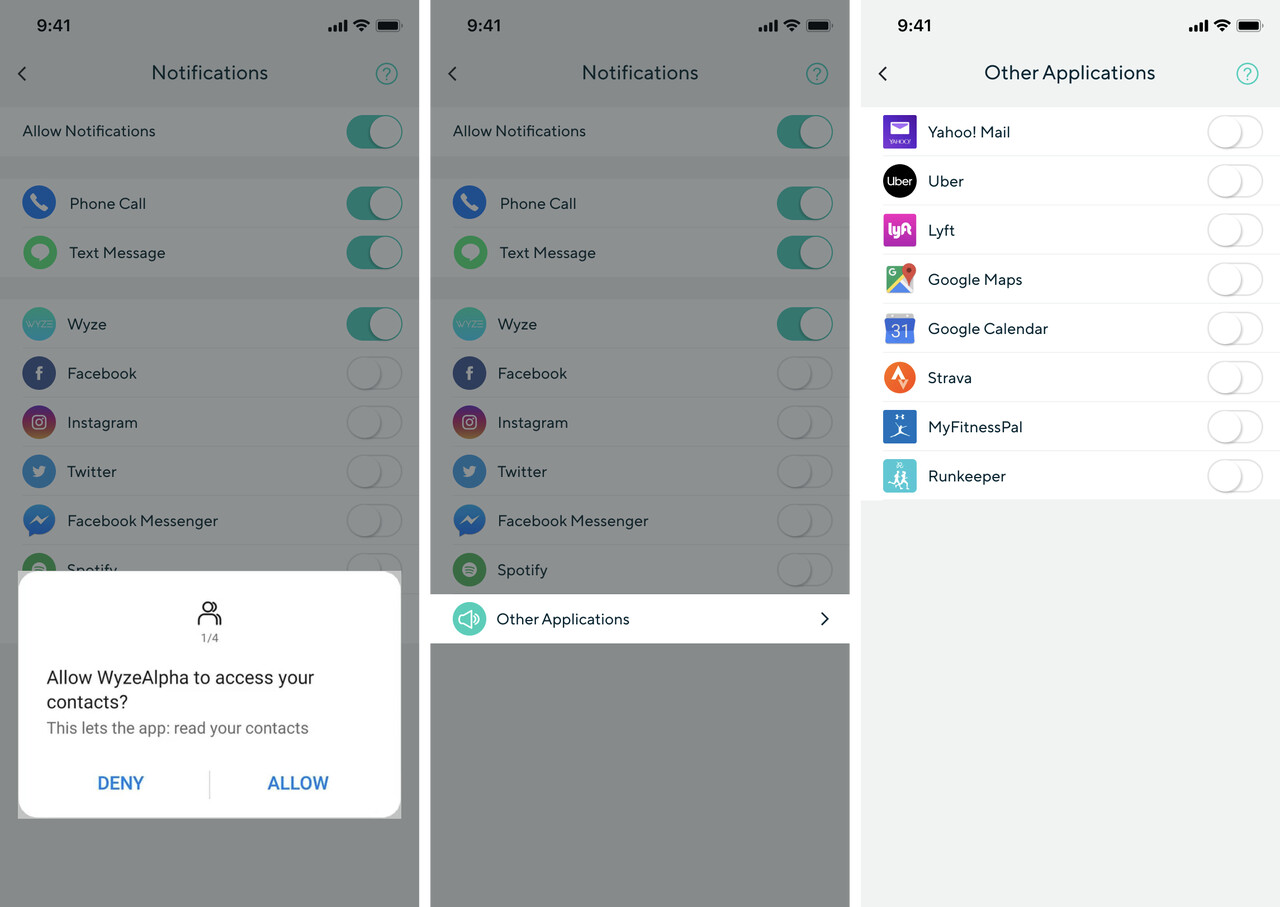**Screenshot Series of a Phone's Notification and Permission Settings**

In this series of three screenshots, we see a detailed view of various settings on a smartphone. Each screenshot captures different ongoing settings and notifications, all organized in a systematic manner.

1. **First Screenshot:** 
   - **Top Section:** The status bar shows typical phone indicators including a phone number (901-941-941), data usage indicators, Wi-Fi signal strength, and battery level icons.
   - **Notifications:** A multitude of repeated notifications are displayed, showing alerts from phone calls, text messages, and popular social media apps like Facebook, Instagram, and Twitter.
   - **Highlighted Apps:** Frequent notifications from Wwise, Facebook Messenger, and Spotify are evident, indicating active or recently used applications.

2. **Second Screenshot:**
   - **Permission Requests:** The focus is on permission settings, with a specific prompt asking whether to allow the app "Wwise Alpha" to access the user's contacts. The options to "Deny" or "Allow" stand out prominently.
   - **Listing of Apps:** Other applications requesting permissions or with pending notifications include Yahoo Mail, Uber, Lyft, Google Maps, Google Calendar, Strava, MyFitnessPal, and Runkeeper.

3. **Third Screenshot:**
   - **Visual Layout:** The two screenshots on the left appear to have a grayish tint, possibly due to lower brightness or a different screen filter applied. This differs from the third screenshot which is more vividly colored.
   - **Content Summary:** Continuation of the app permissions and notifications, with similar apps highlighted again, showcasing a pattern in notification settings and permissions management on this specific device.

This descriptive caption provides a comprehensive overview of the screenshots, detailing the various notification alerts, permission requests, and the visual layout of the phone's interface.